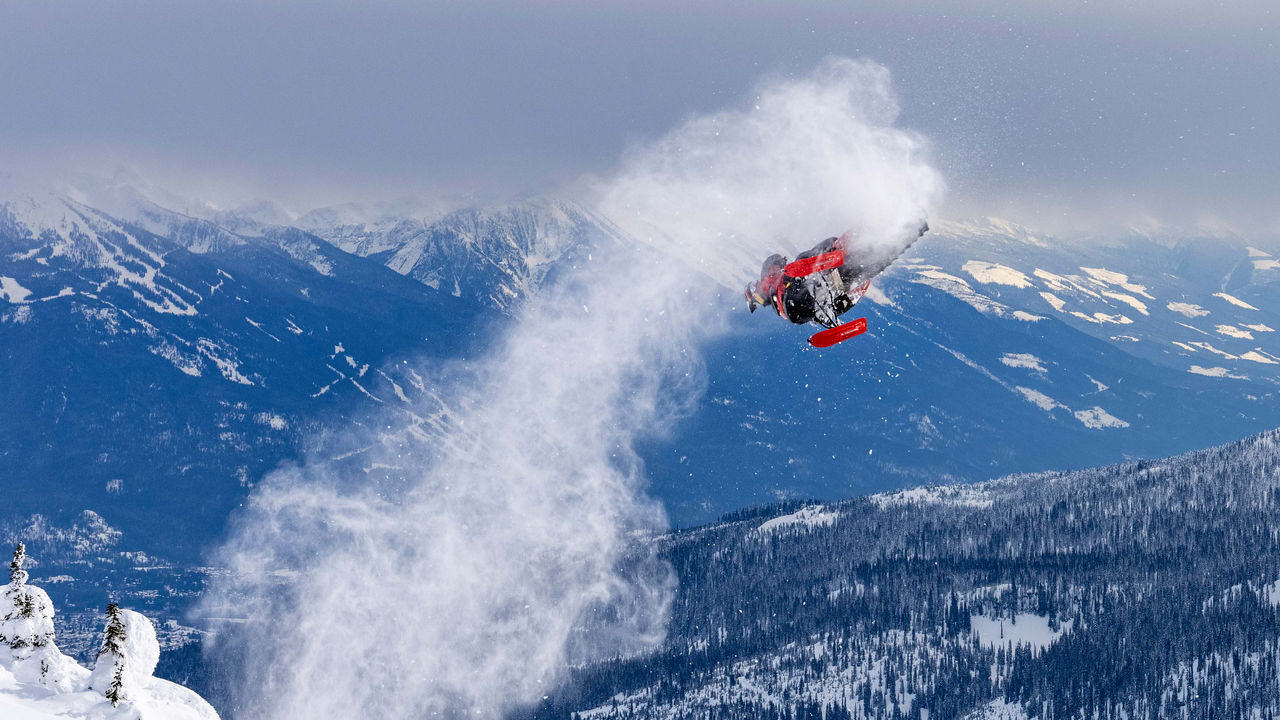The image portrays a breathtaking outdoor winter scene dominated by an expansive blue-hued mountain range with snow-capped peaks. The towering mountains descend into a snowy valley adorned with pine trees. To the right, a smaller mountain, heavily blanketed with snow, features pointy, black pine trees, while to the left, the edge of a hill is visible, also covered with snow and clusters of well-covered pine trees. Dominating the sky is a dramatic cloud of snow dust and smoke, created by a snowmobile performing a high-speed stunt. The rider, dressed in a vibrant red and gray outfit and helmet, is caught mid-flip, with snow trailing off the vehicle's track and tail. This dynamic moment captures the thrill of extreme sports against the serene backdrop of a snowy, mountainous wilderness.